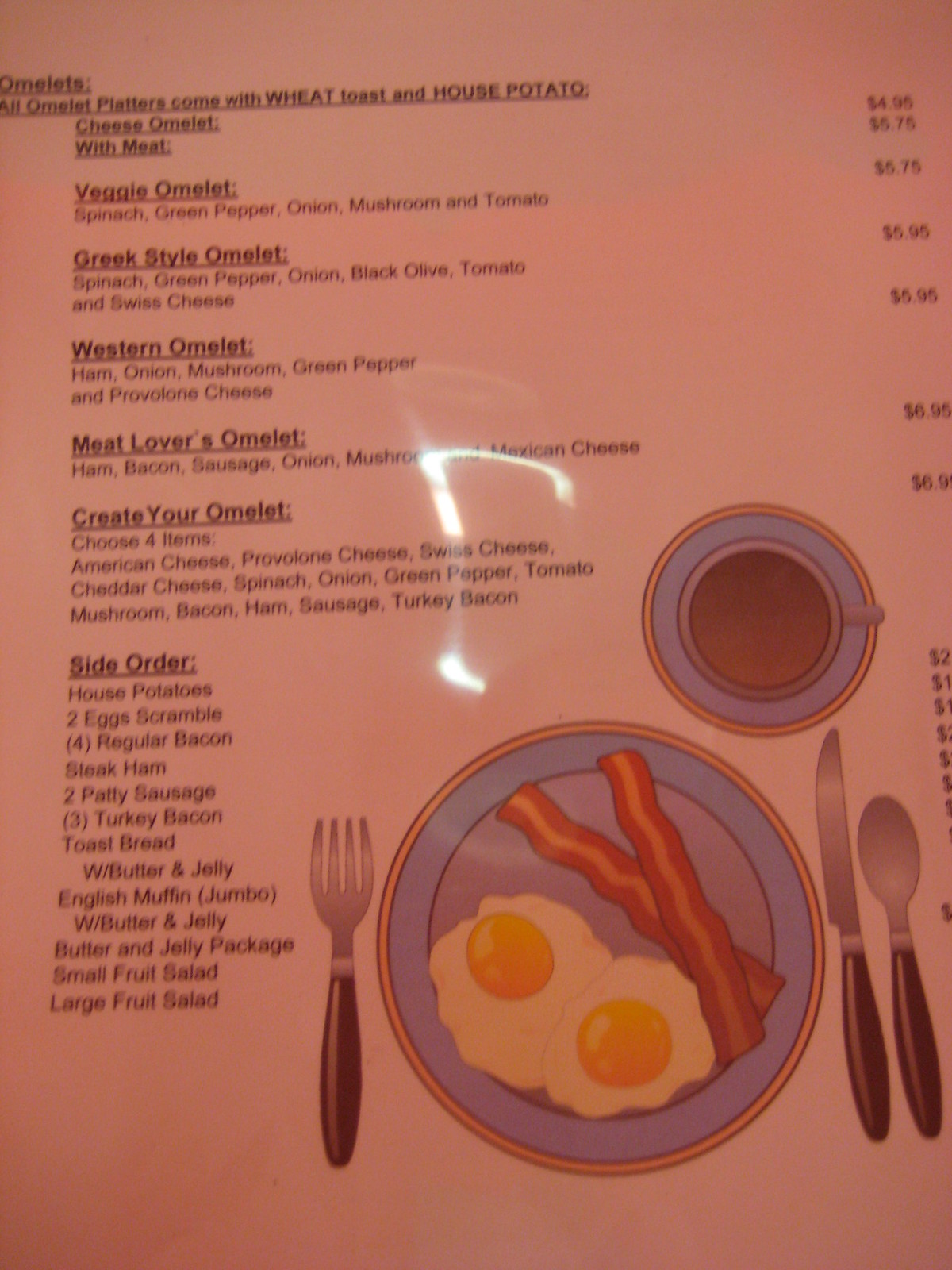The image depicts a rectangular-shaped menu, filling the entire frame, hence no background details of the restaurant, seating, or patrons are visible. The menu has a light source illuminating its center, bordered by a white outline that spans across the top. The menu itself is a peachy salmon color. It appears to display the breakfast section, featuring a graphic resembling a plate with two strips of bacon and two sunny-side-up eggs, outlined in gold, light blue, and dark blue. Accompanying the plate graphic are utensils, with a fork on one side and a knife and spoon on the opposite side, while a coffee mug on a saucer plate is depicted above.

The menu is divided into categories. There is a section dedicated to various omelets including Veggie Omelet, Greek-Style Omelet, Western Omelet, Meat Lovers Omelet, and Create Your Omelet, each accompanied by a description in black text and corresponding prices listed to the side. Below this section, side orders are listed such as House Potatoes and Two Eggs Scrambled, with a detailed description for each item and prices displayed in alignment.